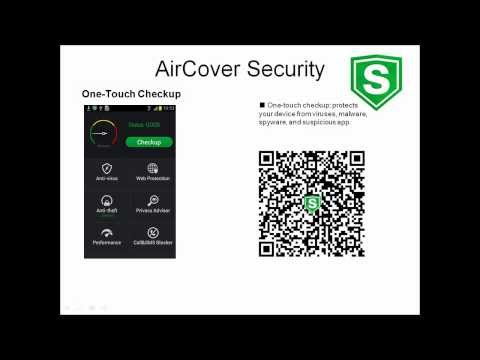The image is a graphic advertisement for Air Cover Security, featuring a black border and a predominantly white background. At the center-top, "Air Cover Security" is prominently displayed. The top right corner showcases the company's logo, a green shield with a white "S" in the middle. 

On the right side of the graphic, a white box contains the text: "One Touch Checkup protects your device from viruses, malware, spyware, and suspicious apps," with a square bullet point preceding the text. Below this text is a QR code, which also has the green shield and white "S" logo at its center.

To the left side of the graphic, there is an image that resembles a screen from a mobile app. The text on this screen reads "One Touch Checkup," and it features several icons: a shield, a magnifying glass, a globe, a padlock, and a leaf. These icons represent different security features, though the text underneath them is mostly illegible, save for words like "web" under the globe and "private" under the magnifying glass.

Overall, this structured layout emphasizes the One Touch Checkup service and its capabilities, while incorporating the brand's distinctive shield logo throughout.